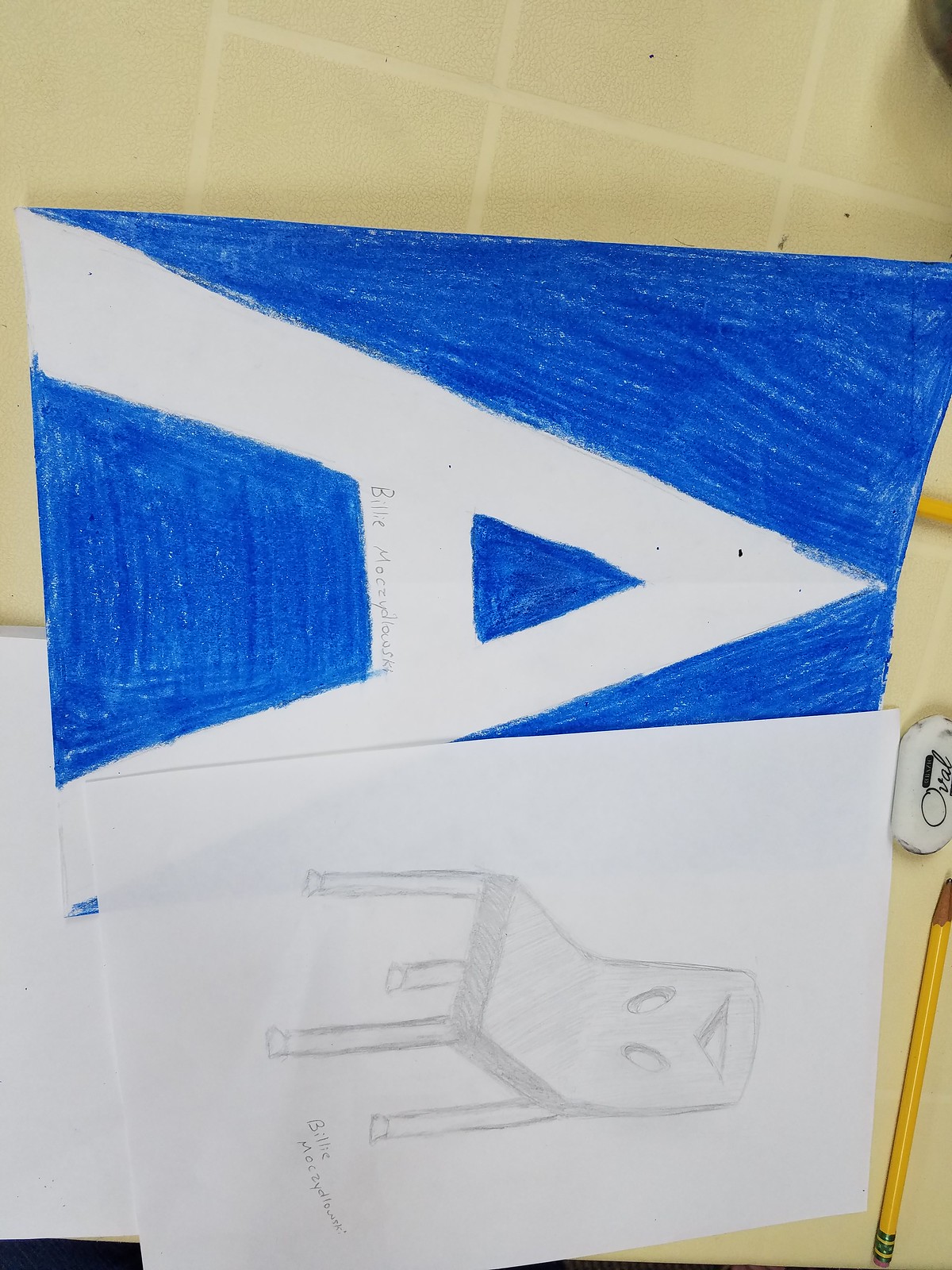The photograph features two pieces of paper showcased on a tan, white-grouted tile surface, angled slightly for added visual interest. A yellow pencil with a graphite tip rests in the lower right corner of the image. The upper piece of white paper prominently displays a large, block letter "A," with a name written below it that is not clearly legible. The background of the "A" is filled in with dark blue marker. Below this, slightly overlapping, is another sheet depicting a pencil-drawn line illustration of a wooden chair. The chair has a straightforward design with four legs and a backrest that includes an upside-down triangle and two oval shapes.